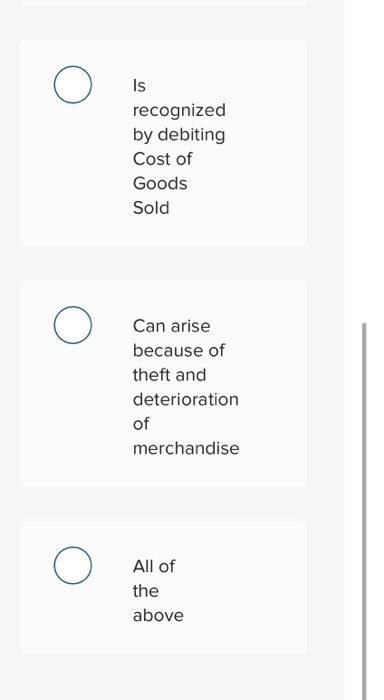A clean and detailed version of that caption might be:

"This is a basic screenshot depicting a multiple-choice question with three possible answers. The layout consists of a long vertical light gray rectangle, divided into three sections, each representing a different option. At the top of each section, there is a smaller rectangle containing text for each option. 

The first option, identified by the statement 'Recognized by debiting Cost of Goods Sold,' is accompanied by a blue open circle on its left side. The second option, located in the middle section, reads 'Can arise because of theft and deterioration of merchandise,' and also features a blue open circle on its left. The third and final option, placed at the bottom, states 'All of the above,' next to another blue open circle. None of the options appear to be selected, as indicated by the open circles remaining unfilled. The text across all options is black, with each line usually containing just one or two words, creating a clean and readable format."